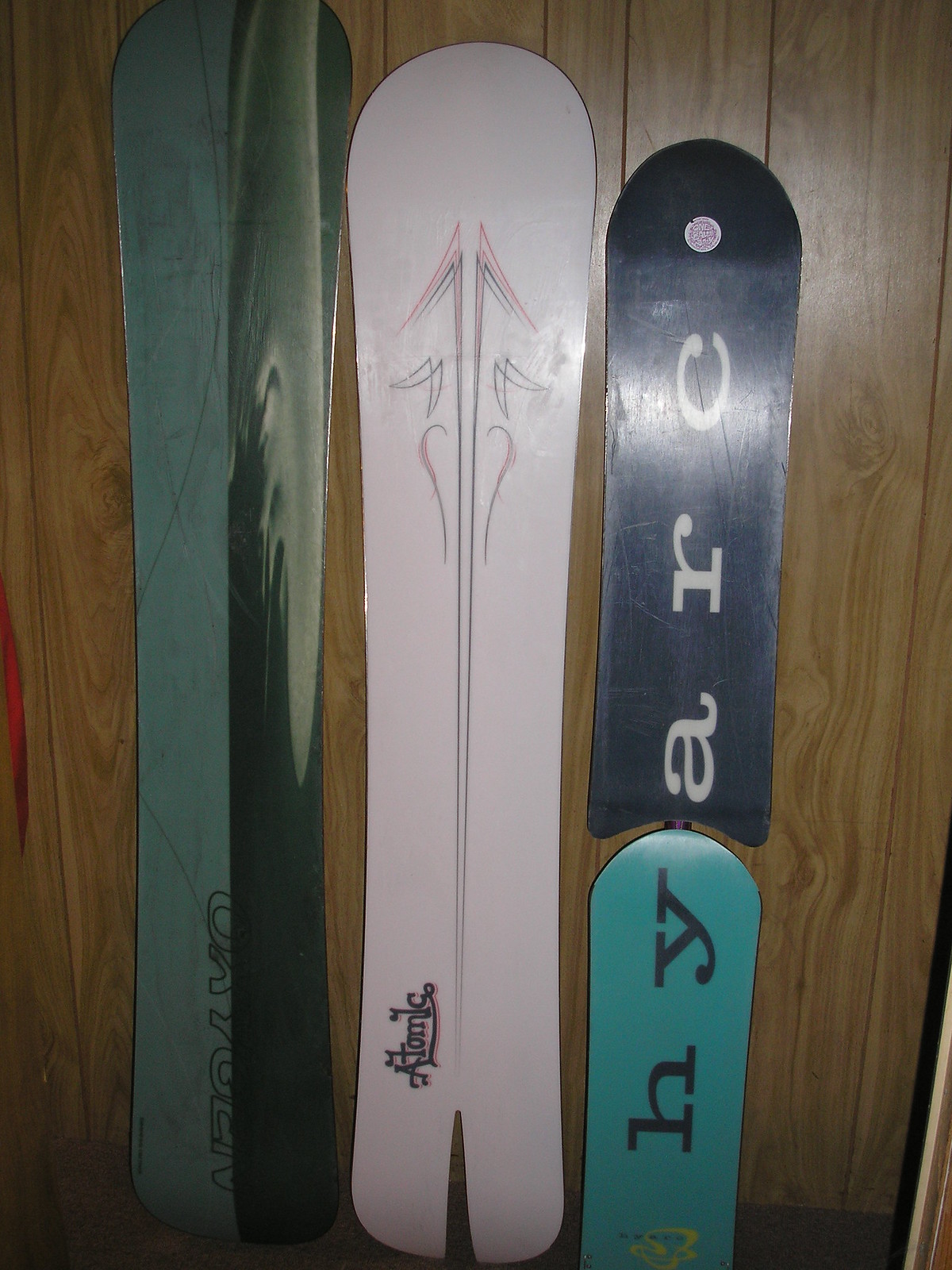In a photograph of a wooden paneled wall, four snowboard decks stand upright, displaying a range of colors and details. On the far left is the tallest board, predominantly green and black, with an indistinguishable word written on it. Next, centrally positioned, is a white snowboard adorned with intricate gray swirl and scroll designs; it features the word "Atomic" in dark lettering on the lower left side. To the right, there are two shorter boards stacked on top of each other. The top board is deep blue with "Arc" written sideways in white letters, while the underlying teal blue board exhibits partial yellow lettering and bold black letters spelling "NY" on its side. The equipment appears to be either mounted on or leaning against the wood paneling, suggesting a cozy indoor setting, potentially someone's home.